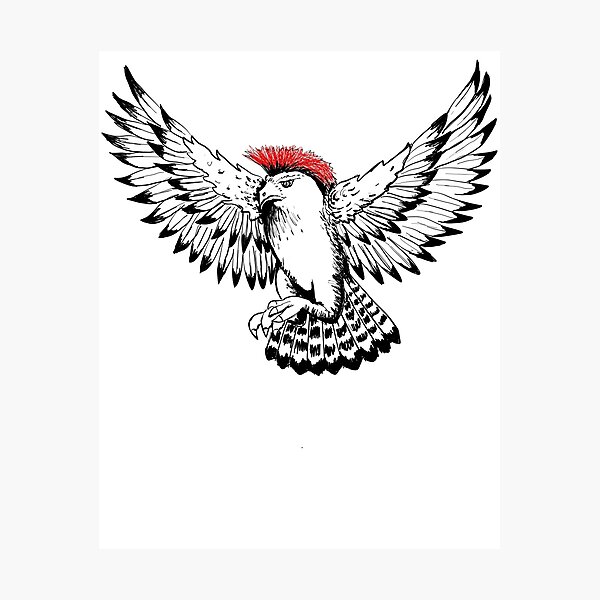This hand-drawn illustration depicts a dynamic bird in mid-flight against a plain white background. The bird, possibly resembling a hawk or an eagle, is primarily rendered in black and white, with striking red feathers forming a mohawk atop its head. Its wings are fully outstretched, displaying three intricate layers of feathers, each detailed with black outlines. The tail feathers point straight down, similarly outlined in black. The bird's talons are raised slightly, drawn in white, and it has a downward-curving beak. The bird is oriented at a 45-degree angle to its right, exuding an intense, almost angry expression. Surrounding the white paper is a light gray background, accentuating the stark, tribal-like design of the image.